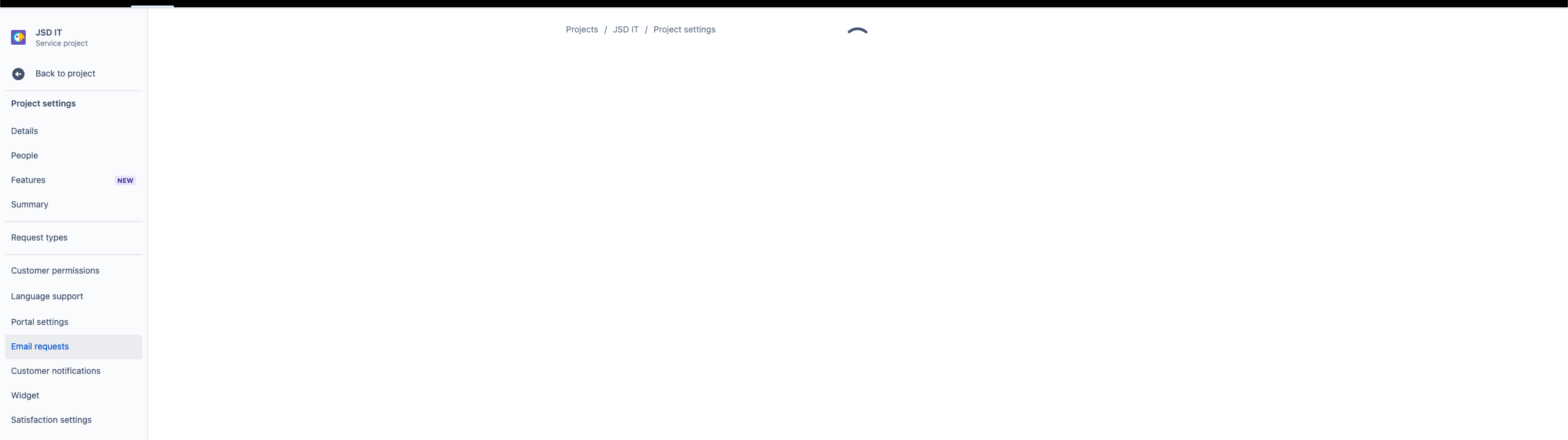The image appears to be a screenshot taken from a computer interface. At the top of the screen, there is a black header that contrasts with the rest of the predominantly white interface. In the upper middle section of the screen, small words are displayed, possibly spelling "JIDIT." Below this header, on the left side, there's a vertical list with numerous items. 

Adjacent to the list, there is a blue square containing a white circle with a touch of orange near its bottom. Adding to the icons, there's a gray circle with a white plus sign inside it, which might be used for adding new items or features. To the left of this, there's another gray circle with a white left-pointing arrow, likely acting as a "Back to Project" button.

Within the list on the left, one item stands out, highlighted with a light gray rectangle around it, indicating it has been selected. The selected item is in blue text, whereas all other items in the list are in gray text.